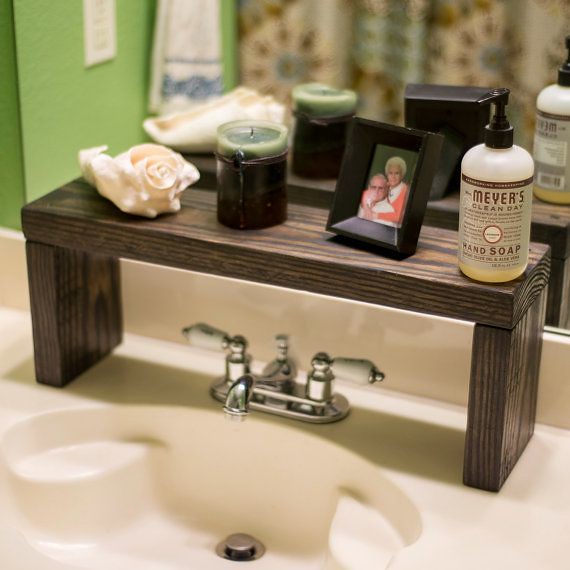In this tranquil bathroom shot, the focal point is a light-colored, possibly cream sink that features a metallic drain and faucet. Above the sink rests a dark wooden stand adorned with an array of carefully arranged items. A large, cream-colored seashell adds a touch of coastal charm, while a green and brown candle invites a soothing atmosphere.

The stand also holds a sentimental photograph framed elegantly; it captures an elderly couple in a warm embrace. The woman, with her short, light-colored hair, wears a white shirt paired with an orange cardigan, her arms lovingly wrapped around the man beside her. The man, possibly sporting glasses, is dressed casually in a white shirt.

Completing the ensemble is a small bottle of Meyers Clean Day hand soap. The soap's packaging transitions from a white upper portion to a yellow base, topped with a practical black dispenser.

The background reveals more of the room's character, with a mirror reflecting the stand and its items, along with a few additional details. You glimpse a softly blurred curtain, green-painted walls, an electrical outlet, and a white and blue towel hanging nearby, rounding out this intimate bathroom vignette.